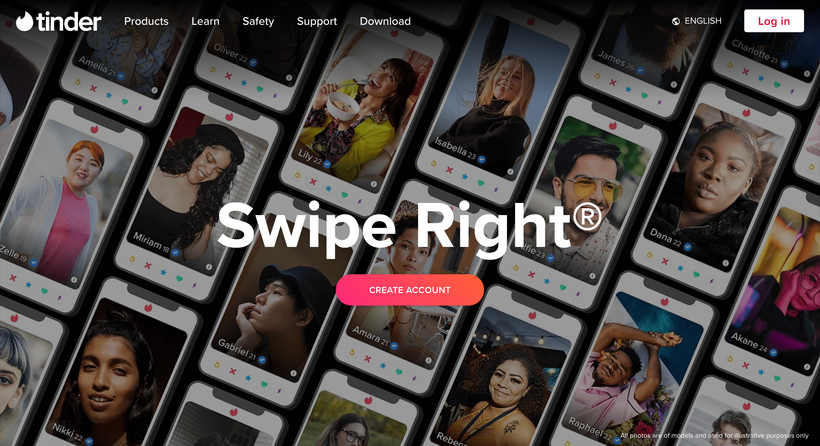The front landing page of the Tinder website, a popular dating app, features a sleek and inviting design. At the top left corner, the Tinder name is prominently displayed in white letters next to its iconic flame logo. Adjacent to the logo, there are navigation options including "Products," "Learn," "Safety," "Support," and "Download." On the opposite end of the top bar, there is an icon of a globe indicating the website is in English, followed by a white "Log In" button with red text.

The background showcases a collage of Apple iPhones, each displaying the Tinder app interface. These iPhones feature various profiles of young men and women, consistent with the app’s purpose of facilitating dating and casual meetups. The largest text on the page invites users to "Swipe Right™," a trademarked slogan synonymous with Tinder’s signature feature. Below this, a prominent "Create Account" button is available for new users.

At the bottom right, there's small, unreadable legal text in white. The profile images of individuals on the displayed iPhones include their first name, age, and a smiling photograph. Each profile offers interaction options such as starring, liking, messaging, or deleting, providing a glimpse into the app's user experience for potential members exploring the site.